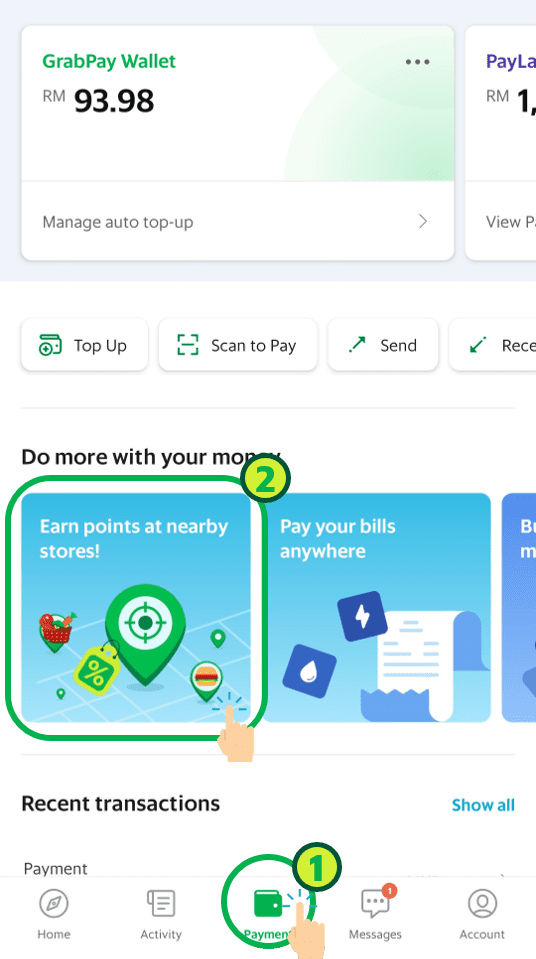This image is a detailed screenshot of a digital wallet app, primarily used for making and receiving payments. The app interface features a clean, white background. At the very top, there's a small window with green text that reads "GrabPay Wallet", displaying a balance of "RM 93.98". Below this, there's an option to "Manage Auto Top Up".

Beneath this top section, a row of four icon-shaped buttons is visible. The first button is labeled "Top Up", the second reads "Scan to Pay", the third says "Send", and the fourth is partially obscured but likely reads "Receive".

Further down, a black-text headline instructs users to "Do More With Your Money". This is followed by three informative windows explaining different functionalities. The first window, highlighted with green text, is labeled "Do" and advises users to "Earn Points at Nearby Stores", accompanied by icons of a map pin and a discount sign. The second window, with light blue text, says "Pay Your Bills Anywhere" and features an icon of a receipt. Unfortunately, the text in the third window is not legible.

Under these informational windows, there is a section titled "Recent Transactions" with an option on the right-hand side to "Show All". 

At the very bottom of the screen, five navigation icons are displayed: "Home", "Activity", "Payment" (highlighted in green with a small notification circle showing the number one), "Messages", and "Account".